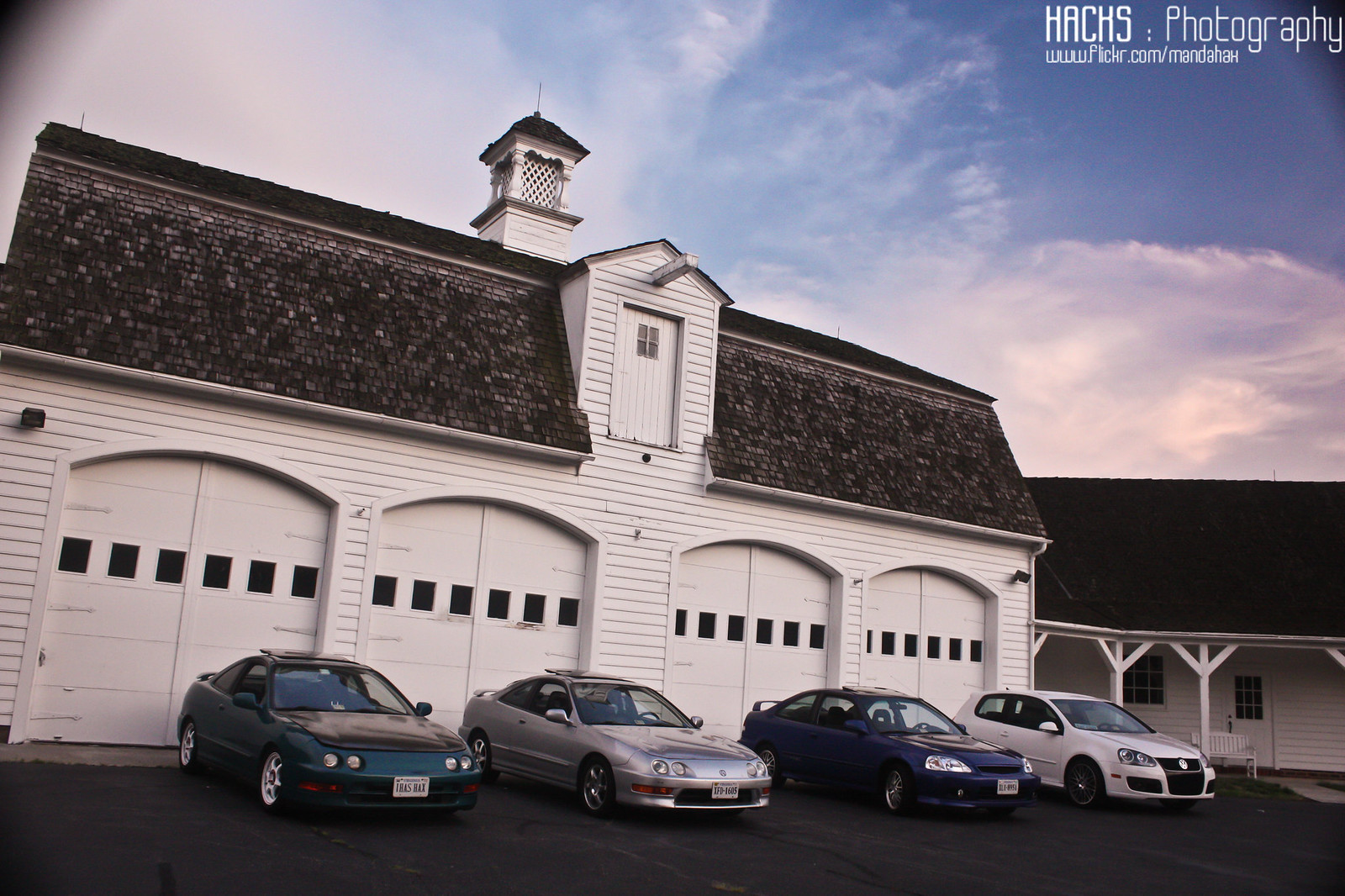This color photograph captures the front of a grand, mansion-like house featuring an expansive quadruple-sized garage with four double-door entrances. Each white garage door, adorned with a row of six small black windows near the top beneath distinctive archways, complements the overall aesthetic of the home's white siding with wooden paneling. The black-tiled roof, speckled with light gray shingles, has prominent smaller structures, including a jettisoned small window and door as well as a detailed spire crowned with white vine-lined pillars tapering off to a dark gray tip. At the house's forefront, four sedans are parked: a bluish-green, a silver, a dark blue, and a white one. The paved driveway extends up to the garage doors, interspersed with a concrete path leading to the house. In the top right corner of the image is the watermark "HACKS Photography", with the web address "www.flickr.com/MandaHah" inscribed below. Black spotlights or security cameras are visible on either side of the main structure, capturing the scene under a blue sky with wispy white clouds. Additionally, the right edge reveals part of another connected house with a white door, black door handle, and white bench, suggesting a complex and well-maintained property.